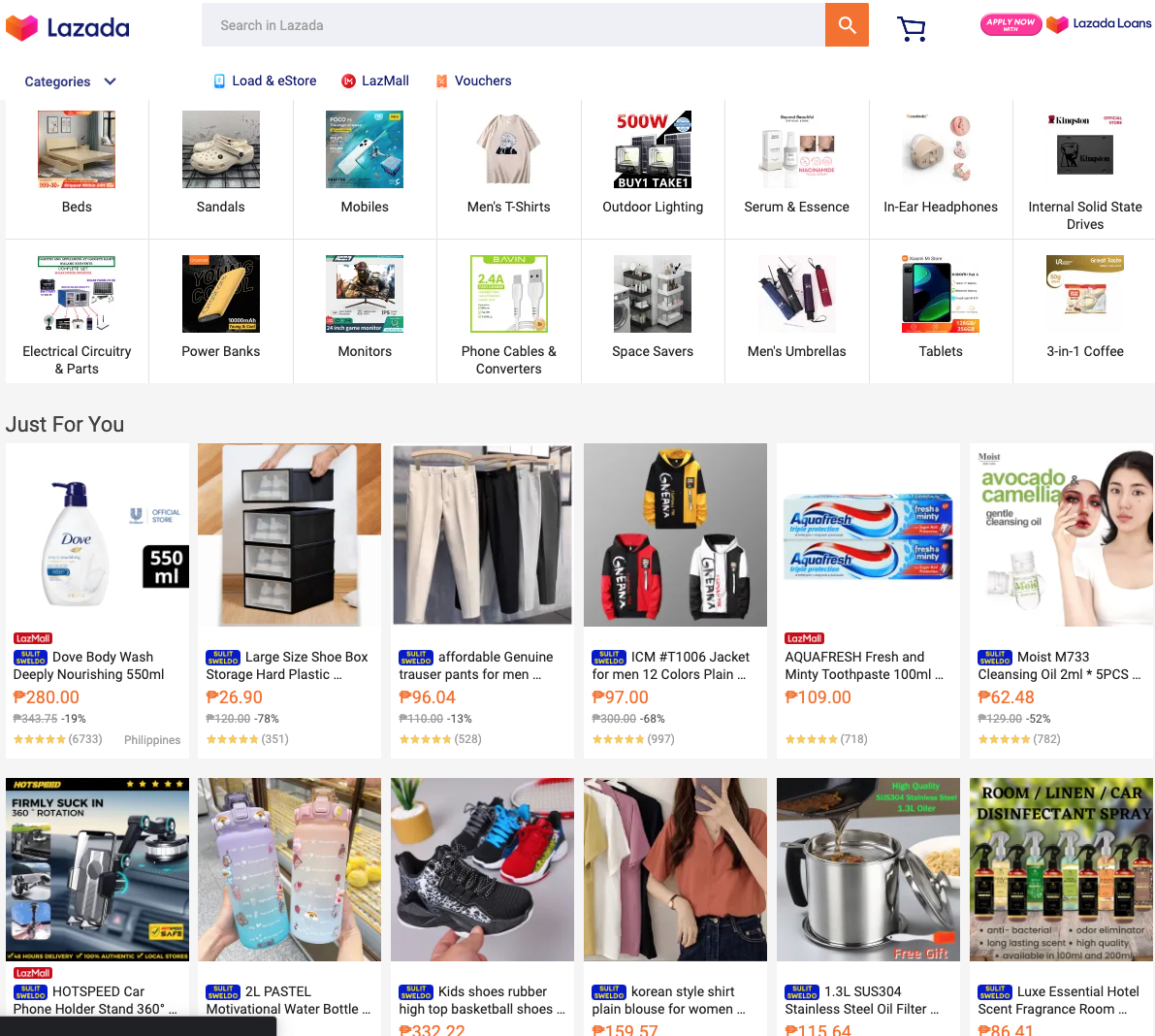In this detailed image of an online shopping website, Lazada, the homepage showcases a diverse array of product categories. At the top, beside the Lazada logo, there is a prominent search bar accompanied by a shopping cart icon. The right-hand corner features a special mention of "Lazada Loans."

The main section of the page displays various product categories, each with representative images. The first row includes items such as beds, sandals, mobiles, men's t-shirts, outdoor lights, serum and essence, in-ear headphones, and internal solid-state drives. 

The following row showcases products like electrical circuitry and parts, power banks, monitors, phone cables and converters, space savers, men's umbrellas, tablets, and three-in-one coffee.

Underneath these, highlighted with images and prices, are items like Dove body wash, large size shoe box, affordable genuine trouser pants for men, jackets for men, Aquafresh fresh and minty toothpaste, moist MZ33 oil, hot speed car phone holder, motivational water bottles, kid's shoes, rubber high-top basketball shoes, Korean-style shirts, plain blouses for women, stainless steel oil filters, and Lux Essential Hotel scent and fragrance room.